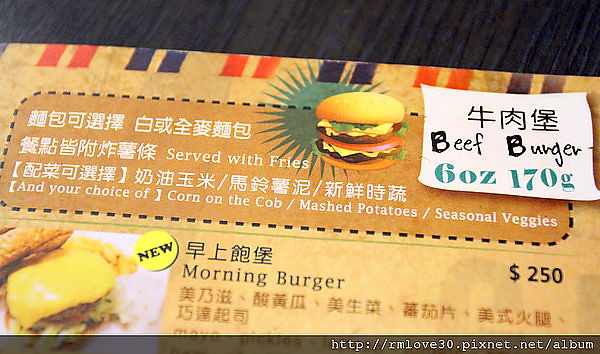The image displays a restaurant menu situated on a dark-colored wood grain table. The menu itself is made of shiny, reflective paper, presenting a tan parchment-textured background. The top of the menu showcases rows of blue and red stripes forming a border. In the center, towards the top, there's a rectangular section outlined with a dotted black line, featuring a darker brown background with a cartoon-like burger in the middle, complete with an orange sunburst behind it. 

The text on this segment of the menu, primarily written in an Asian language—possibly Japanese or Chinese—provides details about the food items. Notably, there's a double patty, double cheese beef burger, garnished with tomato and lettuce, described as "beef burger, 6oz, 170g" and labeled as "morning burger" priced at $2.50. Additionally, a section mentions the meal is served with fries and offers a choice of sides including corn on the cob, mashed potatoes, and seasonal veggies. At the very bottom right of the image, there is also a URL: "http://rmlove30.picsnet.net/album." All these elements combined depict a comprehensive snapshot of a vibrant, international burger menu.